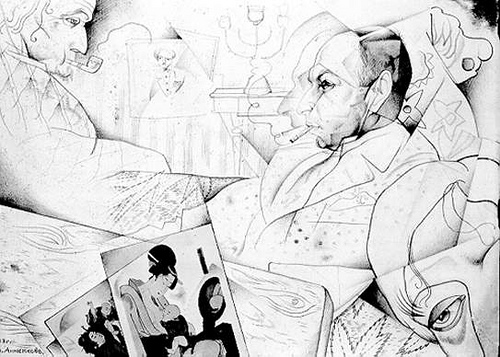This black-and-white abstract sketch, likely created with pencil or pen, depicts a scene with three men arranged within a room. Dominated by shades of gray, the image places most objects and people near the top. On the left side, a man faces right, identifiable by his pipe, prominent nose, and right eye. Another man, closer to the foreground, faces left with a cigarette in his mouth, and his left eye and nose are visible, along with the lapel of his jacket. In the extreme foreground at the bottom right, a right eyeball peers into the scene, suggesting another person's presence very close to the viewer. Toward the bottom of the image, a table hosts a few photos, one clearly depicting an Asian woman with other pictures in a similar style. Between the men in the background, a candelabra or Hanukkah candle adds to the room's detailed ambiance. The overall composition, reminiscent of a comic book, lacks any textual elements and focuses instead on the intricate, monochromatic interplay of objects and figures.